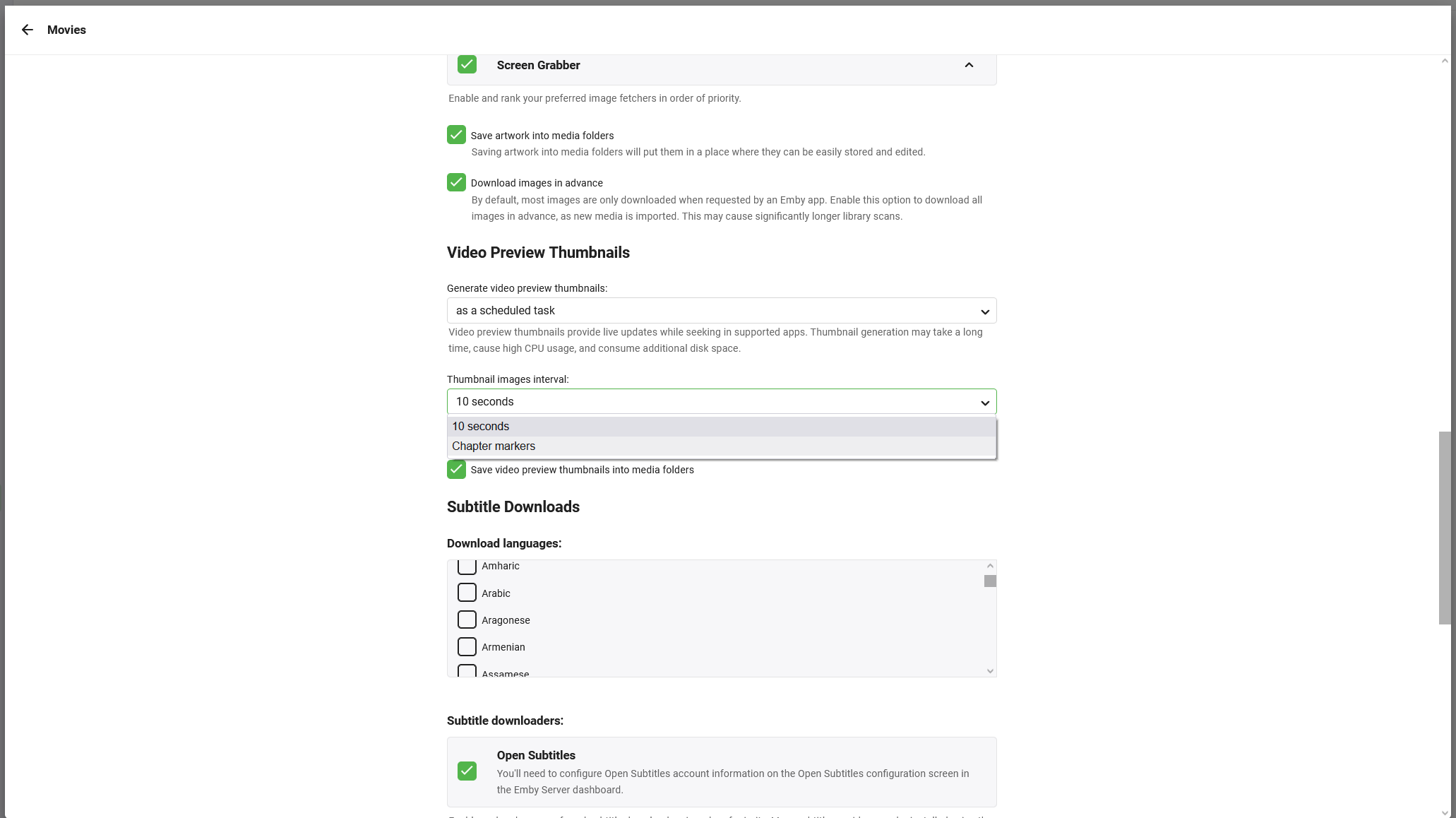The image appears to be a web page dedicated to the submission of a video, possibly for a platform similar to YouTube, though it does not exactly resemble YouTube's interface. At the top of the page, there are several check boxes, one of which, labeled "screen grabber," is checked. Two additional check boxes are present below this section, but the details are difficult to discern due to the small text.

Beneath these check boxes is a header titled "Video Preview Thumbnails," followed by a scroll box containing the text "Shareable." Just below this scroll box, there is yet another check box.

Further down the page, a header titled "Subtitle Downloads" is displayed. Under this heading, there is a list of languages available for subtitle download, each accompanied by a corresponding check box. Notably, the option for "Open Subtitles" is checked.